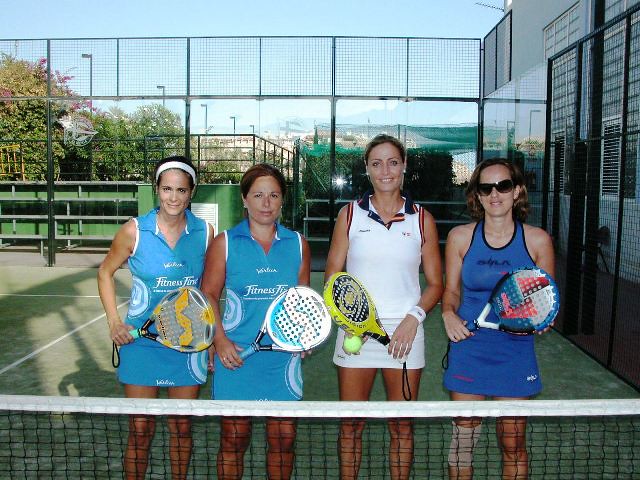The photograph captures a moment on a tennis court featuring four middle-aged women, each holding tennis rackets, standing behind a net with a white top border. The court is green and appears to be made of a turf material. 

Starting from the left, the first two women are dressed in matching teal v-neck tanks and skirts, with the first woman also sporting a white sweatband. The woman to her right holds a gray and yellow racket, while the next one has a white and blue racket. The third woman, taller than the others, is dressed in a white v-neck tank and skirt, holding a yellow and black racket in one hand and a tennis ball in the other. The woman on the far right dons a dark blue tank and skirt, complemented by sunglasses, and grips a white, blue, black, and red racket.

Behind them, there are tall fences and lighting posts surrounding the tennis court. The background features a clear blue sky with some greenery, possibly trees, visible to the top left. A glass or metal enclosure is hinted at, reflecting the daylight which casts some shadows on the court. The women are smiling, looking forward, encapsulating a moment of camaraderie and shared enjoyment on the court.